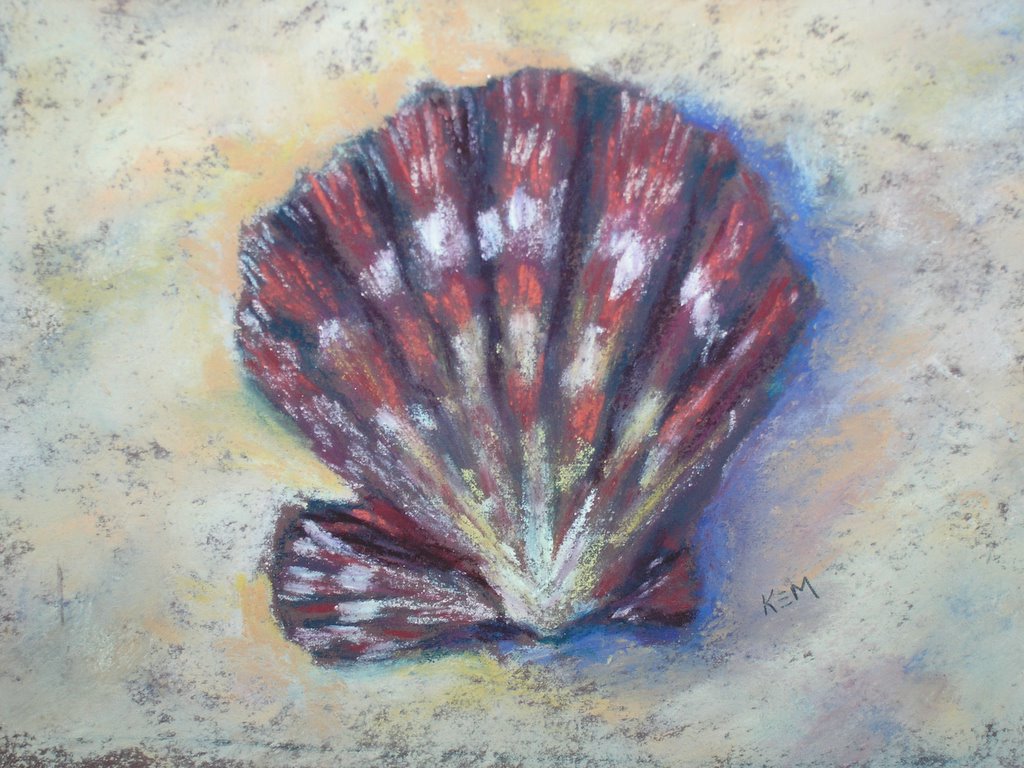The painting presents a large, vibrant seashell centrally positioned against a sandy, beach-inspired background. The seashell, dominating the middle third of the image, is vividly painted in striking hues of red, white, orange, and yellow. The top portion boasts a deep red, transitioning below into alternating sections of white and orange, culminating in yellow and white at the bottom. The shell appears fan-shaped, pointing towards the top of the painting, with intricate detailing showing eight parts on top. The background evokes a beach setting, with light beige sand in the left and right areas, accented by streaks of blue, peach, and smoother white, creating the appearance of wet and dry sand layers. A subtle blue shading frames the shell, enhancing its prominence. On the bottom right, the inscription "K-E-M" is noticeable, adding a personal touch to the piece. The surrounding sandy area is speckled with small dots of white, orange, and black, contributing further texture to the scene.